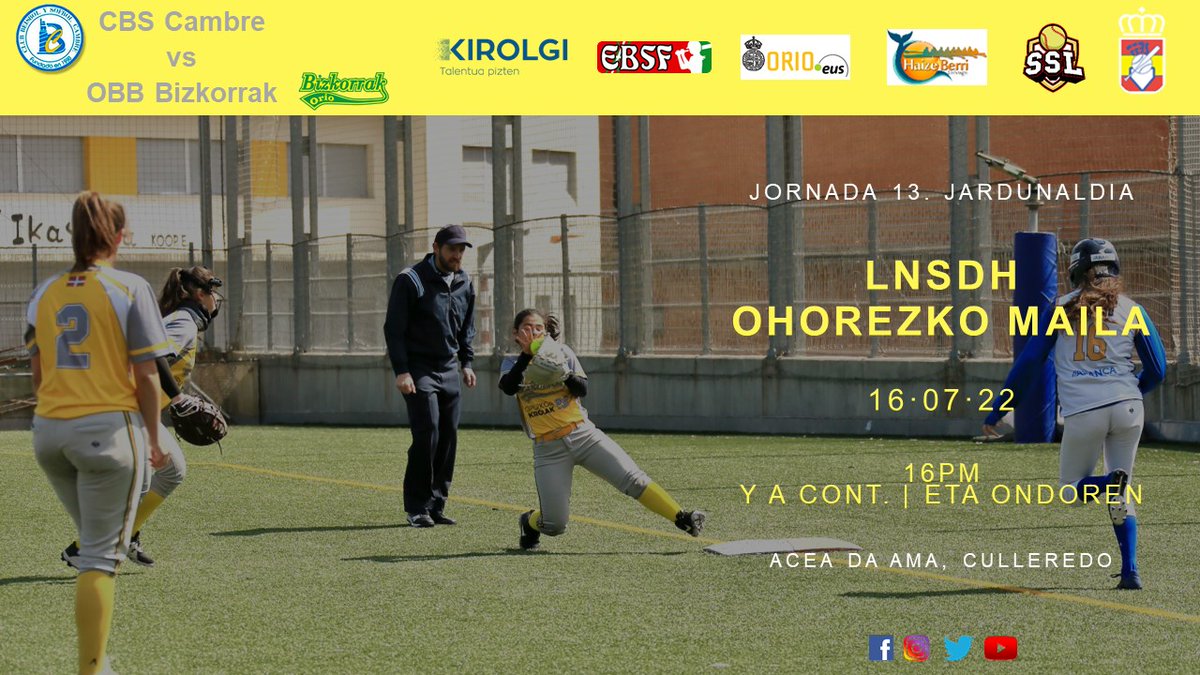The image is a rectangular photograph, measuring approximately three to four inches tall and six inches wide. It prominently features a girls' softball game taking place outdoors on a sunny day. The main focus is on a dynamic moment where one of the girls in a yellow and gray uniform is in the midst of catching a ball near a base, while a girl in a blue and gray uniform, wearing the number 16, is running toward that base.

At the top of the image, there is a yellow header stretching across the entire width, adorned with various sponsor logos. On the left, there is a white circle with a blue letter "B" inside it, outlined in blue. Next to it in gray print is "CBS, Camber versus OBB, BizCorac," and in red lettering "BizCoract." Further right in blue print is "Koroge," followed by a logo with a red background and white print reading "EBSF." Continuing along, there is a white rectangle with yellow print that reads "ORIO" and in black print "EUS." Next, another white rectangle features an image of a sun and what appears to be a whale's tail with the name "Hasbury." The subsequent logo depicts a shield with a baseball and the initials "SSL" in white print. Finally, on the far right, there is a red and gold shield with a baseball bat and a white crown on top.

On the right-hand side of the image, in white print, are the words "Jornada 13" and "Jardinaldia." Below this, in yellow print, it reads "LNSDH" and "OHOREZKOMAILA." Further below, the date "16.07.22," the time "16 p.m.," and the location "YACONT E-T-A-O-N-D-O-R-E-N" are displayed. Additionally, in white print, it says "ASEA DE ALMA CULEREDO." The bottom of the image features logos for Facebook, Twitter, Instagram, and YouTube, indicating the presence of social media links.